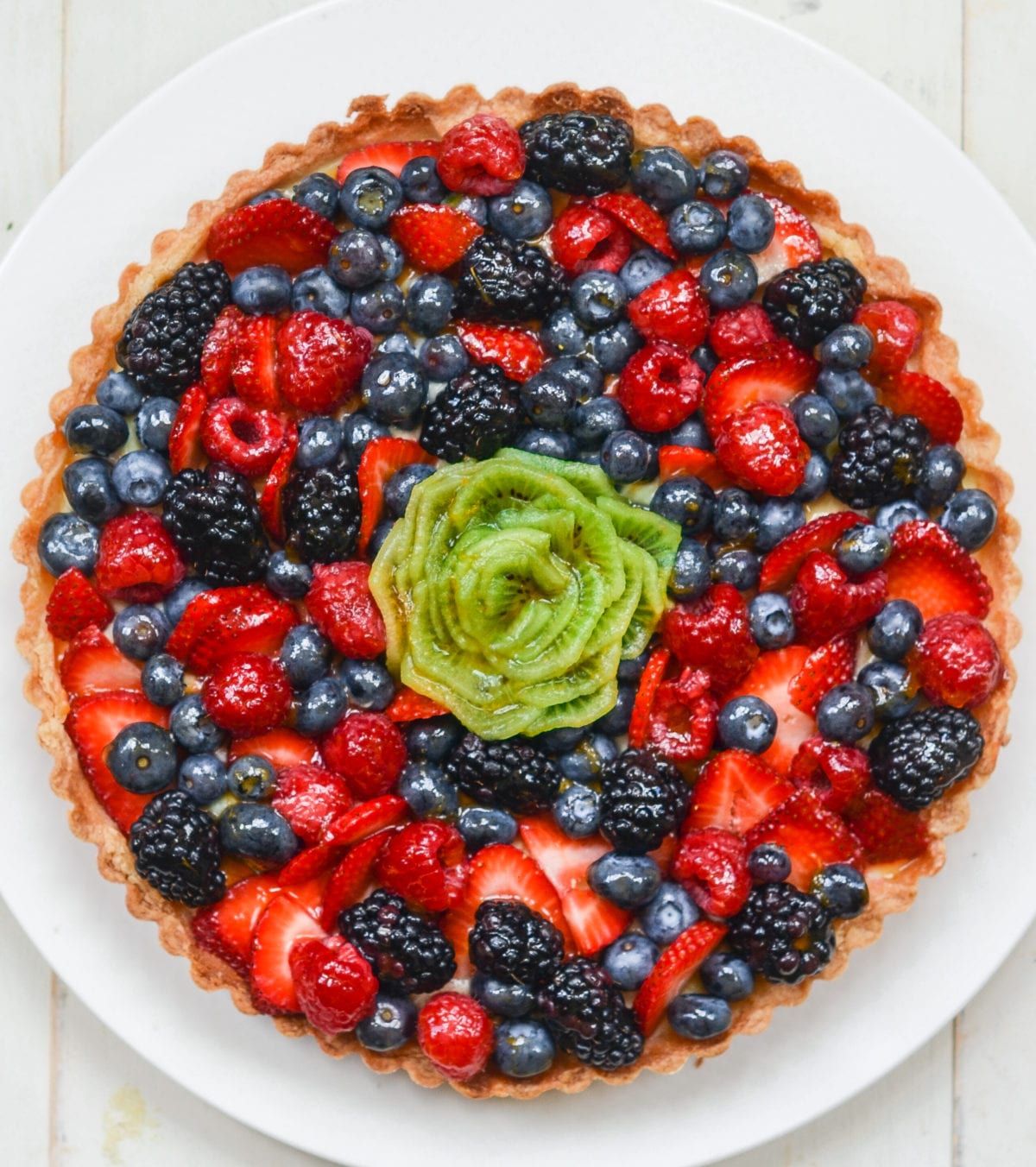This close-up indoor photograph captures a tantalizing berry tart, perfectly presented on a white plate set atop a white wooden table. The table shows a slight stain at the bottom left-hand side, adding a touch of rustic charm to the scene. The round tart features a beautifully crimped, golden-brown traditional pie crust that is scalloped along the edges. The crust exhibits an inviting variance in brown shades, indicating a well-baked finish.

The tart itself glistens, hinting at a light glaze covering the fresh assortment of summer berries. Sliced strawberries, plump blueberries, juicy blackberries, and vibrant raspberries are artfully arranged around the outer edge. At the center of this delightful creation is an exquisite rose made from delicate slices of kiwi, adding an artistic and fresh green touch to the dessert.

The plate's edges are slightly cut off on the left and right sides of the photograph, emphasizing the tart as the focal point. There are no utensils or additional elements visible in the image, allowing the beauty of the tart to stand alone. Despite the simple backsetting, the rich, natural colors of the berries—red strawberries, blue blueberries, black blackberries, and red raspberries—stand out vividly against the pristine white plate and table. This untouched, glossy berry tart appears delectably fresh and ready to be served at a party or dinner, inviting anyone who sees it to take the first slice.